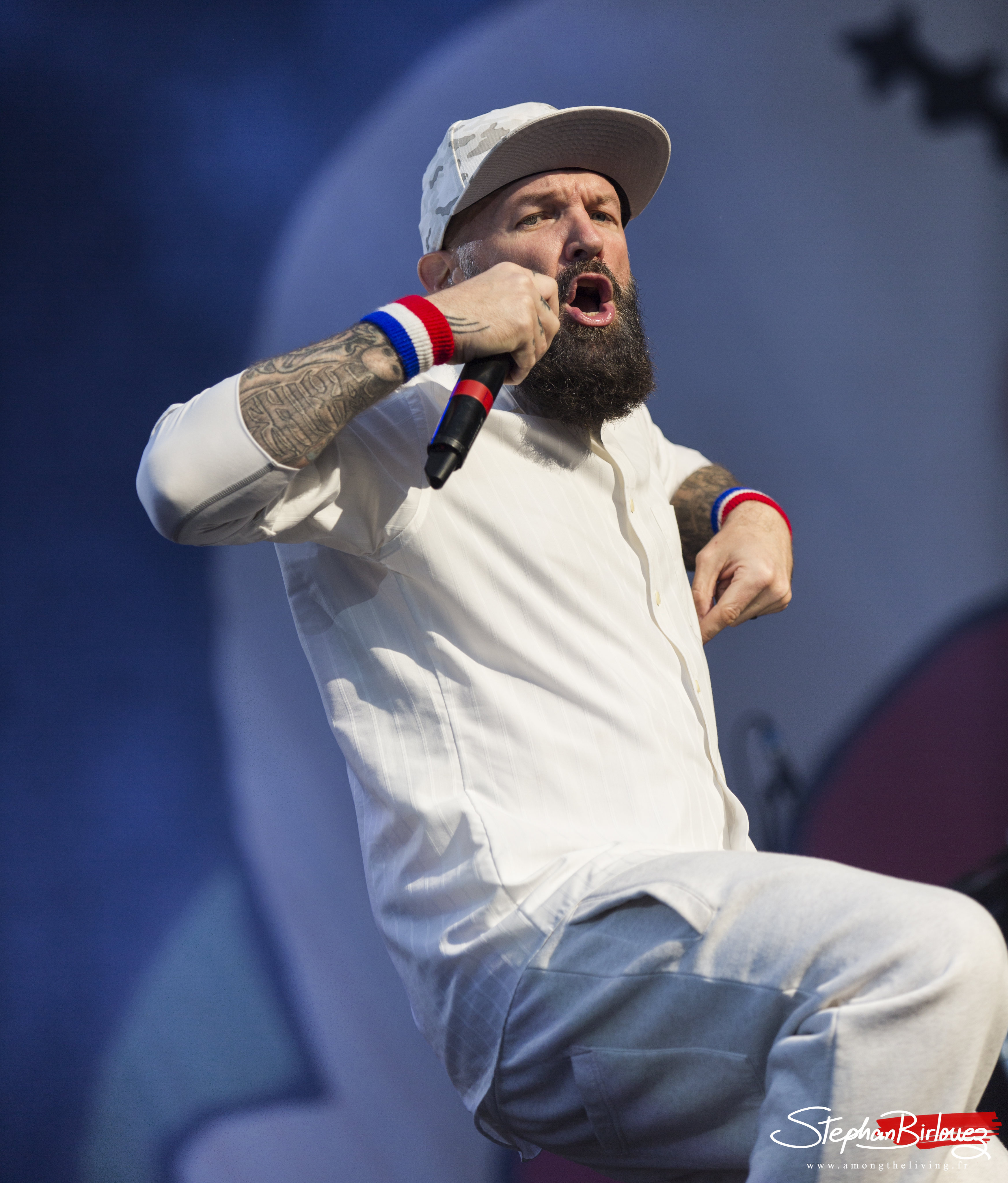This photograph captures a dynamic side view of a large white man, mid-performance on stage. He is dressed entirely in white, featuring a white cap, a buttoned-up shirt with mid-length sleeves, and pale-colored jeans. His visible arm is adorned with tattoos, one of which appears to be a female figure, and he sports a red, white, and blue wristband reminiscent of the French flag. His thick black beard and mustache frame his open mouth as he sings passionately into a black microphone with a red stripe. The background vividly displays a mix of white, blue, and red hues, complementing the vibrant energy of his stance, which suggests he is either walking or dancing. Notably, at the bottom right corner of the image, the name "Stephen Birloi" is written in white text.